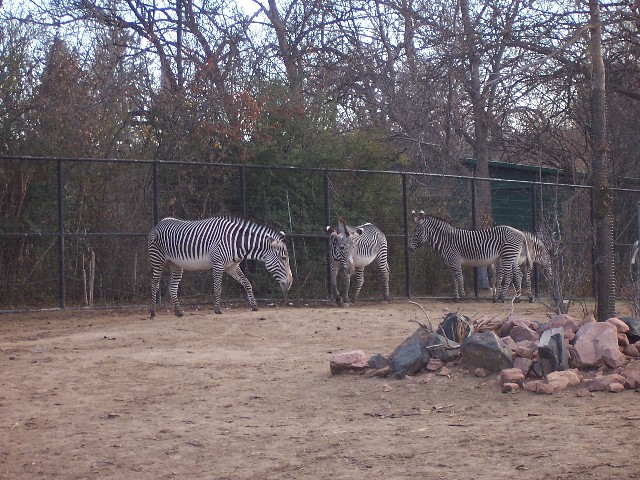This image captures a small group of four zebras in a zoo enclosure, seeming to move or stand with heads held high and one front foot raised, suggesting a walking motion. The zebras are in captivity, evidenced by the tall black chain-link fence that rises about twice the height of their backs. Beyond the fence, there is thick vegetation comprising leafless trees, shrubs, and a dark green building that partially emerges from the greenery. The foreground of the enclosure is characterized by bare, light brown dirt, with a cluster of rocks and a tree positioned on the right side. The scene hints at an autumn setting, with some leaves in the trees appearing brown, adding to the dull, slightly drab atmosphere of the enclosure.